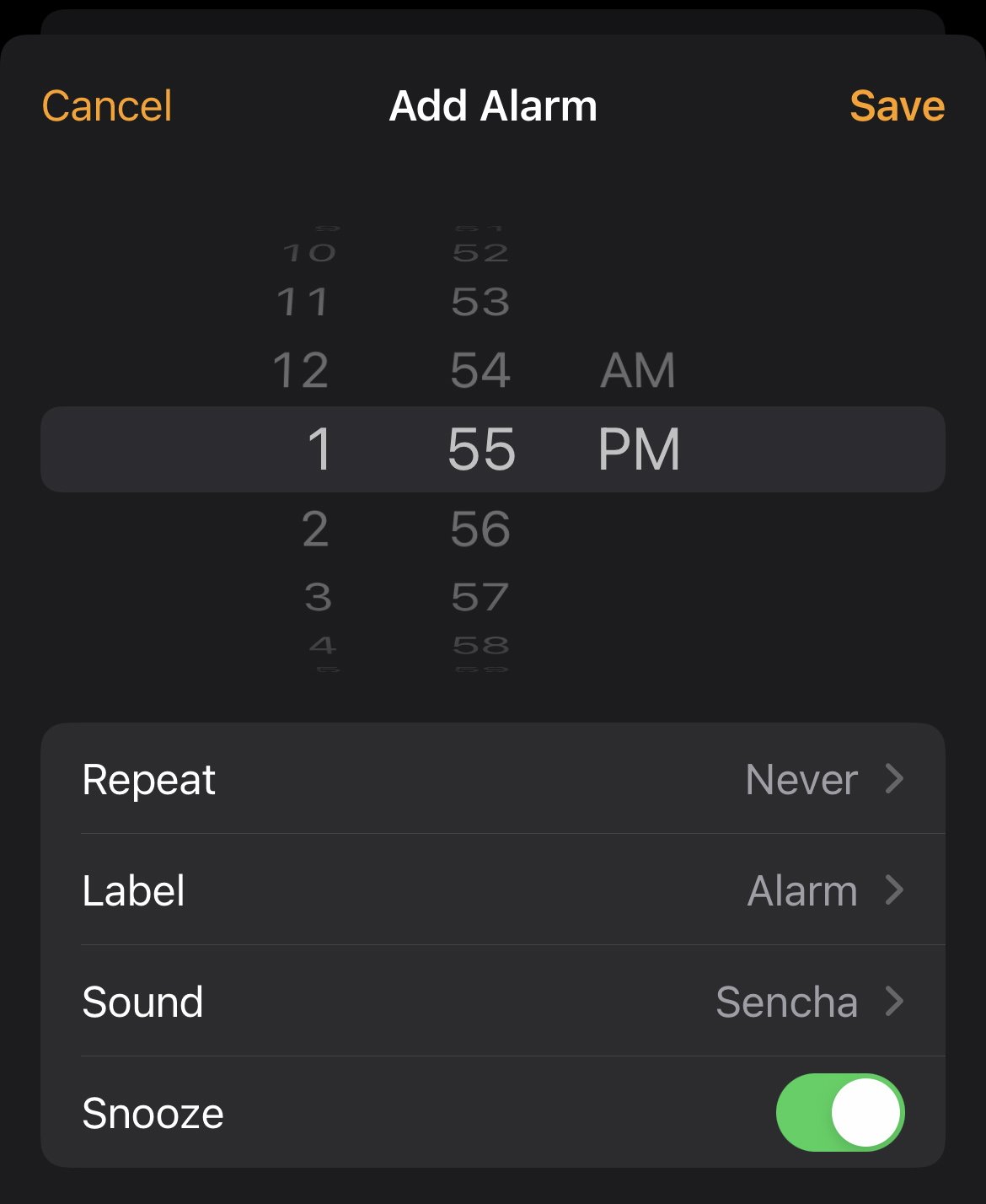**Screenshot Description of a Mobile Alarm Setup Interface:**

This detailed screenshot captures a mobile phone's alarm setup interface. At the top of the screen, there is a white text header labeled "Add Alarm." On the left-hand side of the screen, a button labeled "Cancel" appears in an orange-yellow color, allowing the user to cancel the alarm setup process. On the right-hand side, a "Save" button, also in an orange-yellow color, is present for saving the configured alarm.

Below the header, the time setting interface is displayed. It consists of three vertically arranged columns. The first column, which is for selecting the hour, is highlighted with the number "1." The second column, designated for minutes, is highlighted with "55." The third column allows the user to switch between "AM" and "PM," with "PM" currently selected in capital letters.

Further down, there are several categorical options available:

1. **Repeat:** This option currently displays "Never" with a small arrow beside it, indicating further options can be explored by tapping it.
2. **Label:** This option has the default label "Alarm" and an arrow to customize the alarm label.
3. **Sound:** This category shows "Default Sound" with an accompanying arrow, suggesting that the user can select different alarm sounds.

Lastly, there is a **Snooze** option featuring a toggle switch. The snooze function can be turned on or off by sliding the button left or right. When enabled, the toggle switch appears green with a white dot.

The comprehensive layout is user-friendly and provides a complete overview for setting up and customizing the alarm according to personal preferences.